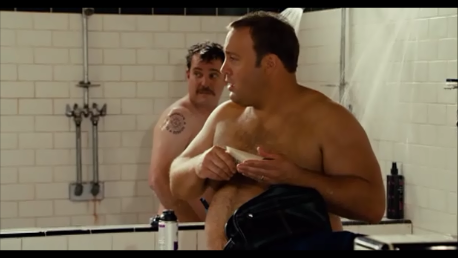The image depicts actor Kevin James, shirtless, standing in a shower scene with another shirtless man slightly behind him and to his left. Kevin, rotund with very short hair, holds a bar of soap while both men look towards the left of the frame, as if something has caught their attention. The white tiled wall in the background and visible plumbing fixtures suggest a bathroom setting. The water is running from the showers, and a black bottle, possibly shampoo, sits on a counter to the right of Kevin's elbow. Both men are partially obscured, with the second man's arm visible but less prominently featured. The photo is horizontal and rectangular, likely a promotional or movie scene.